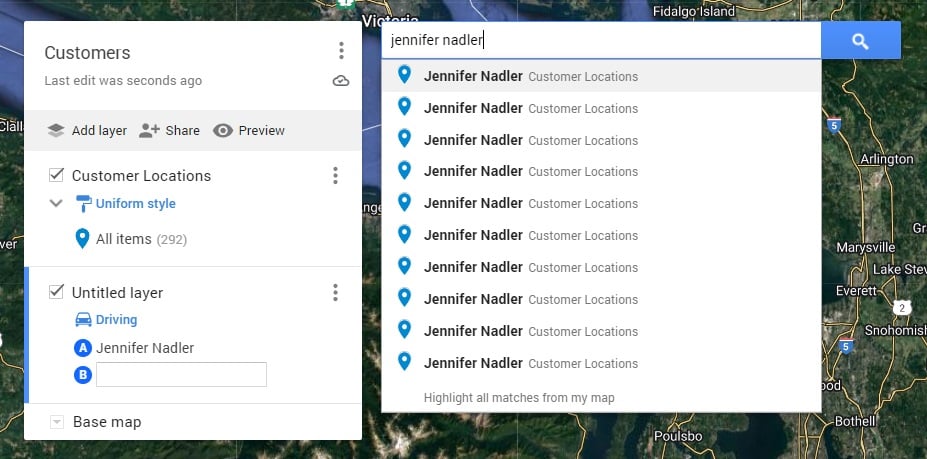The image is a detailed screenshot of a digital map with a focus on the area around the Great Lakes. The map prominently displays regions such as Victoria, Fidalgo Island, Arlington, Marysville, Lake Stevens, Everett, Snohomish, Bothell, and Poulsbo, marked in blue to indicate water bodies. 

On the left side of the image, there's a white sidebar containing several options and details. It reads: "Customers last edited seconds ago," with options including "add layer," "share preview," "customer locations," and "uniform style," which depicts a paint roller icon. Below these options, it specifies "all items: 292" and "untitled layer," marked by a blue car icon representing "driving." Additionally, the text mentions Jennifer Nadler and other users in an input field.

At the top-right corner of the map, a white search box shows the name "Jennifer Nadler" typed in, with a blue search button on the right adorned with a magnifying glass icon. The search results manifest in a drop-down menu with around ten items, each marked by a location pin and labeled "Jennifer Nadler customer locations." The drop-down concludes with a selectable option to "highlight all matches from my map."

This comprehensive screenshot effectively captures both the geographic region displayed and the user's interactive options within the map interface.